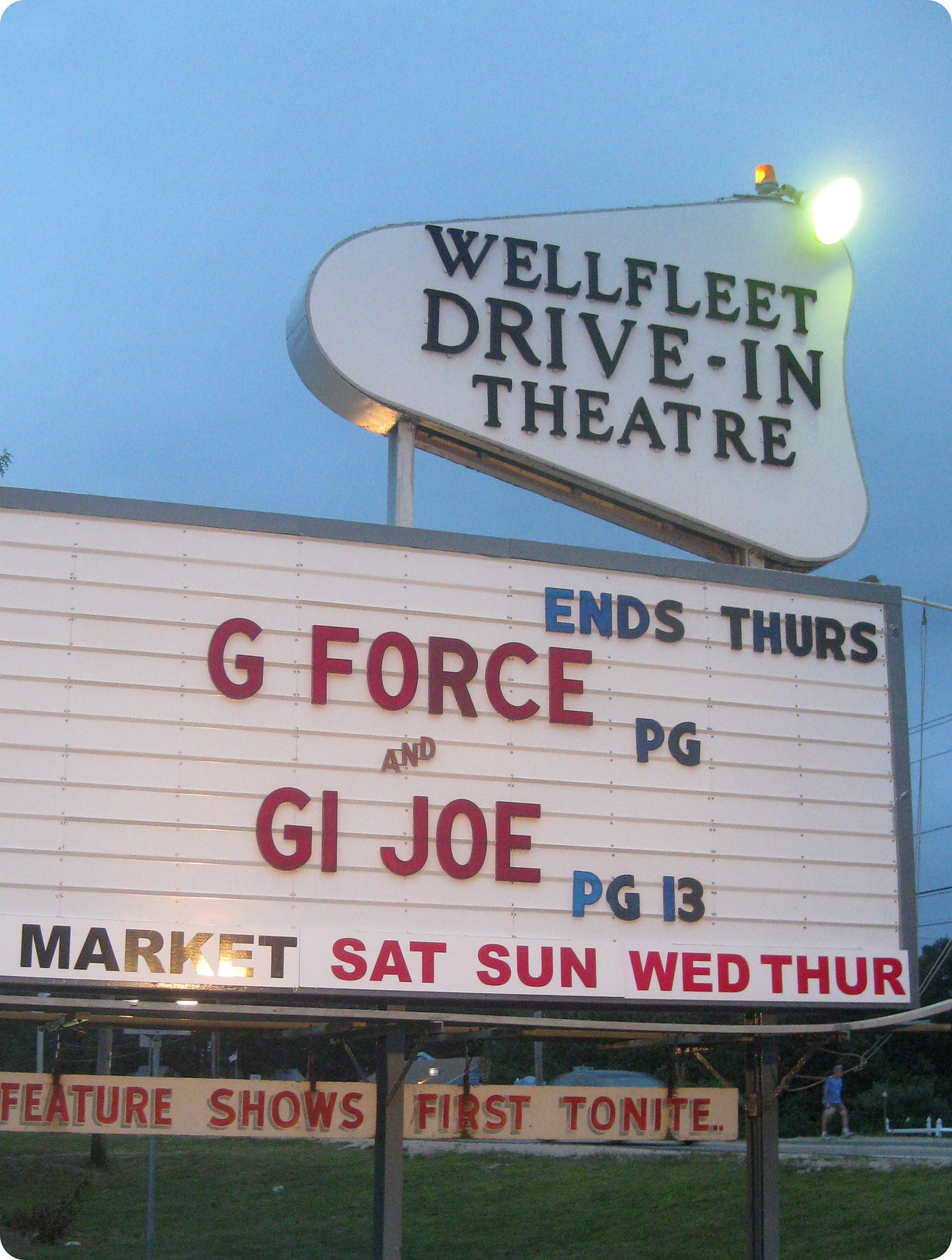The photograph captures a Wellfleet Drive-In Theater sign prominently displayed in the center of the image. The sign comprises two stacked sections, with the top section featuring a rounded arrow shape with black lettering that reads "Wellfleet Drive-In Theater." Below, the larger rectangular section has a white background with blue text stating "Ends Thurs." In red text, the films "G-Force" rated PG and "G.I. Joe" rated PG-13 are listed. "Market" is written in black lettering, followed by the days "Sat, Sun, Wed, Thur" in red. Two smaller panels hang beneath with yellow backgrounds and red text, indicating "Feature Shows First Tonight."

A grassy area extends below the sign, blending into the background where a man in a blue shirt and black shorts is seen walking on a road, slightly blurred. The scene is set against a twilight sky that is beginning to darken. A yellow spotlight illuminates the sign, emphasizing its details. The photograph effectively showcases the drive-in theater's offerings and the surrounding environment.